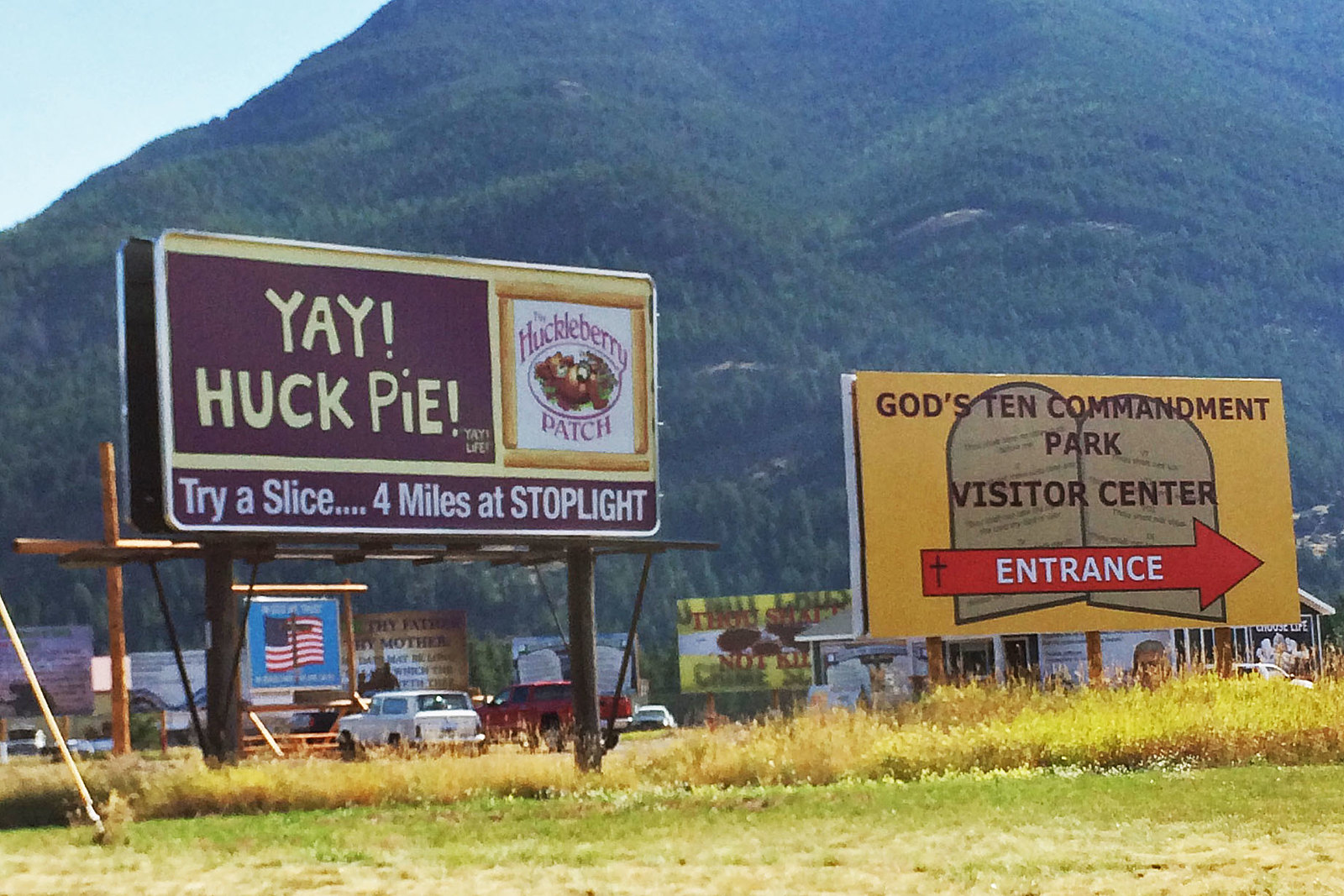In this photograph, taken in a lush, forested area, two prominent billboards stand against a backdrop of a tall hill covered with trees. The foreground features a vibrant green field where multiple cars are parked around the billboards. 

The first billboard, located on the left, captures attention with its playful graphic of a bear lounging on its back with arms behind its head. This sign promotes the "Huckleberry Patch" and features a cheerful text bar next to the bear that reads, "Yay! Huck Pie! Try a Slice! Four Miles at Stoplight."

Adjacent to it, the second billboard contrasts with its more solemn gold background, displaying two arching stone tablets. This billboard invites visitors to the "God's Ten Commandments Park Visitor Center," with an eye-catching red arrow pointing towards the entrance.

Together, the billboards create a juxtaposition of playful and religious imagery set within the tranquility of a forested environment.